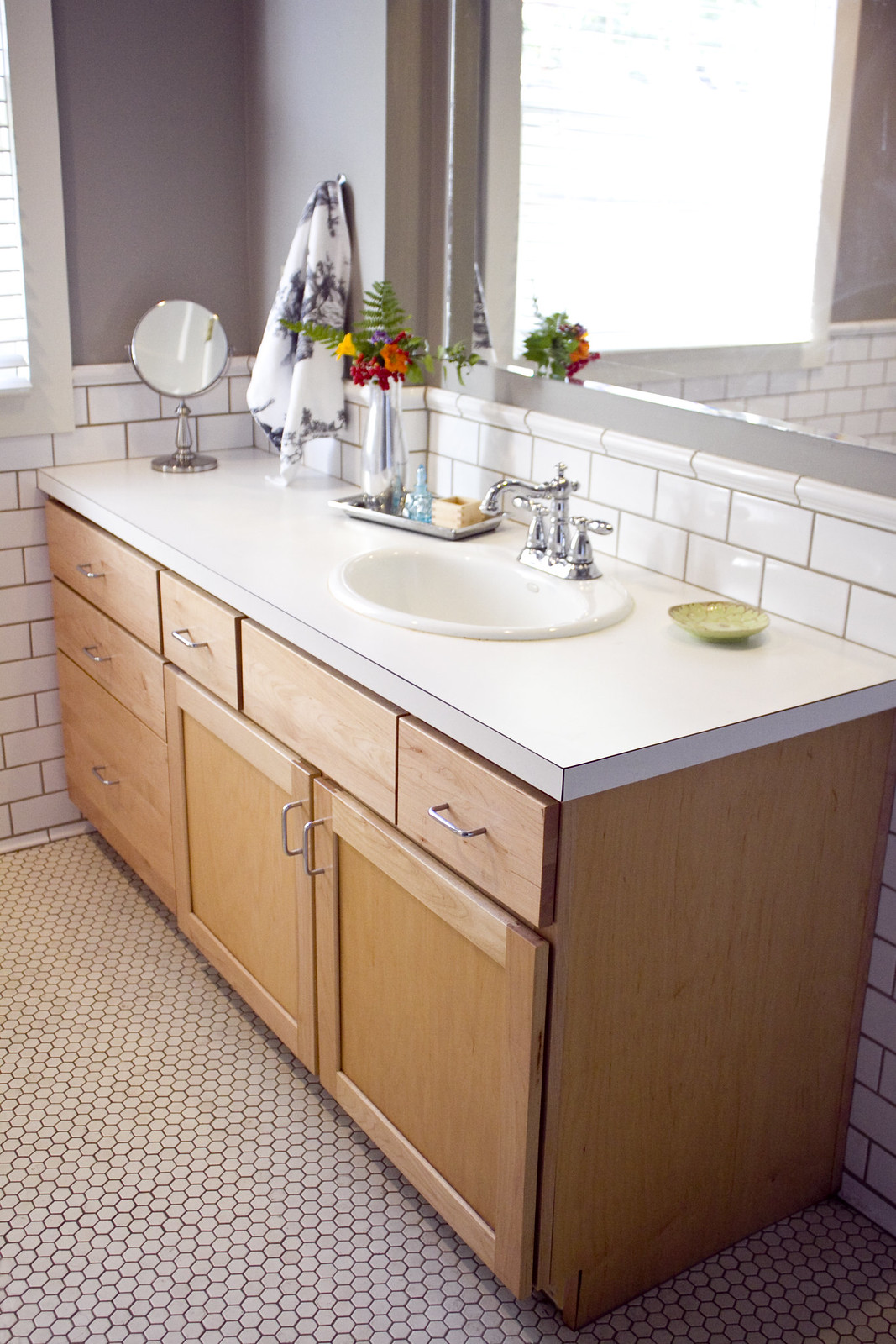This photograph showcases a modern bathroom captured in portrait mode. The sink countertop features pristine white Formica, complemented by a light wood vanity base with slender, silver handles. The vanity extends horizontally with numerous drawers and includes two cabinets below the sink area. The shiny silver faucet stands out against the backdrop of rectangular white tiles that rise about a foot above the sink. Adornments on the countertop include a vase brimming with fresh flowers, a green soap dish, and a round stand mirror with a silver finish. A stylish towel, patterned in white and black, hangs neatly on the wall. The upper section of the wall is painted in an elegant shade of gray, further enhancing the bathroom's contemporary aesthetic.